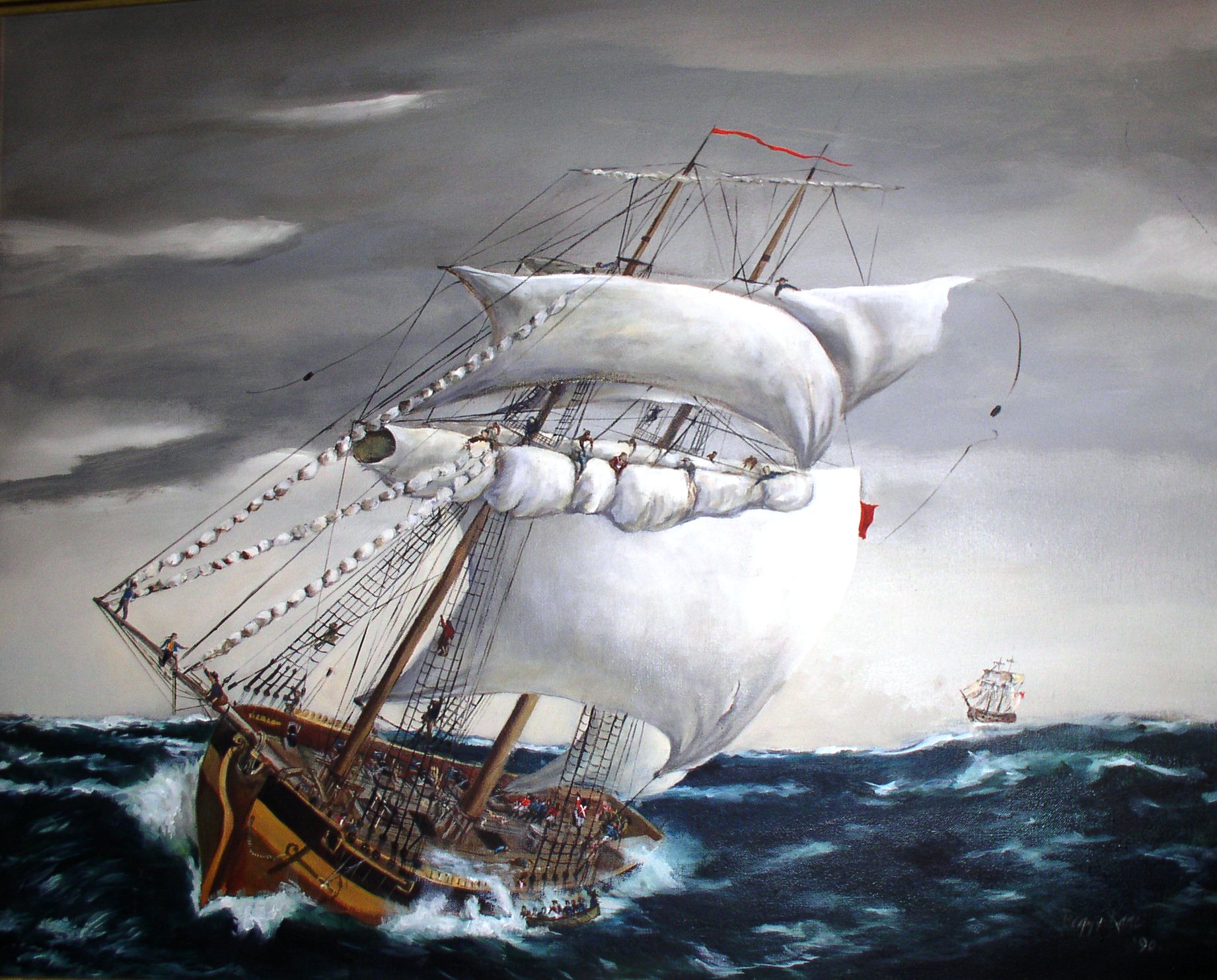This painting portrays a dramatic scene of an older ship battling rough seas, tilted dangerously to its side as if on the verge of capsizing. The ship is adorned with large white sails and features a small red flag at the top of the mast, accompanied by another smaller red flag slightly lower. Amidst the chaos, several crew members climb the ropes, seemingly striving to adjust the sails and stabilize the vessel. The tumultuous sea swirls around them, while water spills through the ship’s holes, hinting at the imminent danger. Off to the left in the far distance, a second, smaller ship is visible. Meanwhile, the lifeboat is being deployed with crew members attempting to climb aboard. The scene is intensified by the dark, gray sky filled with ominous rain clouds. The artist's name is inscribed in the lower right corner, though it is small and faded, rendering it difficult to read.